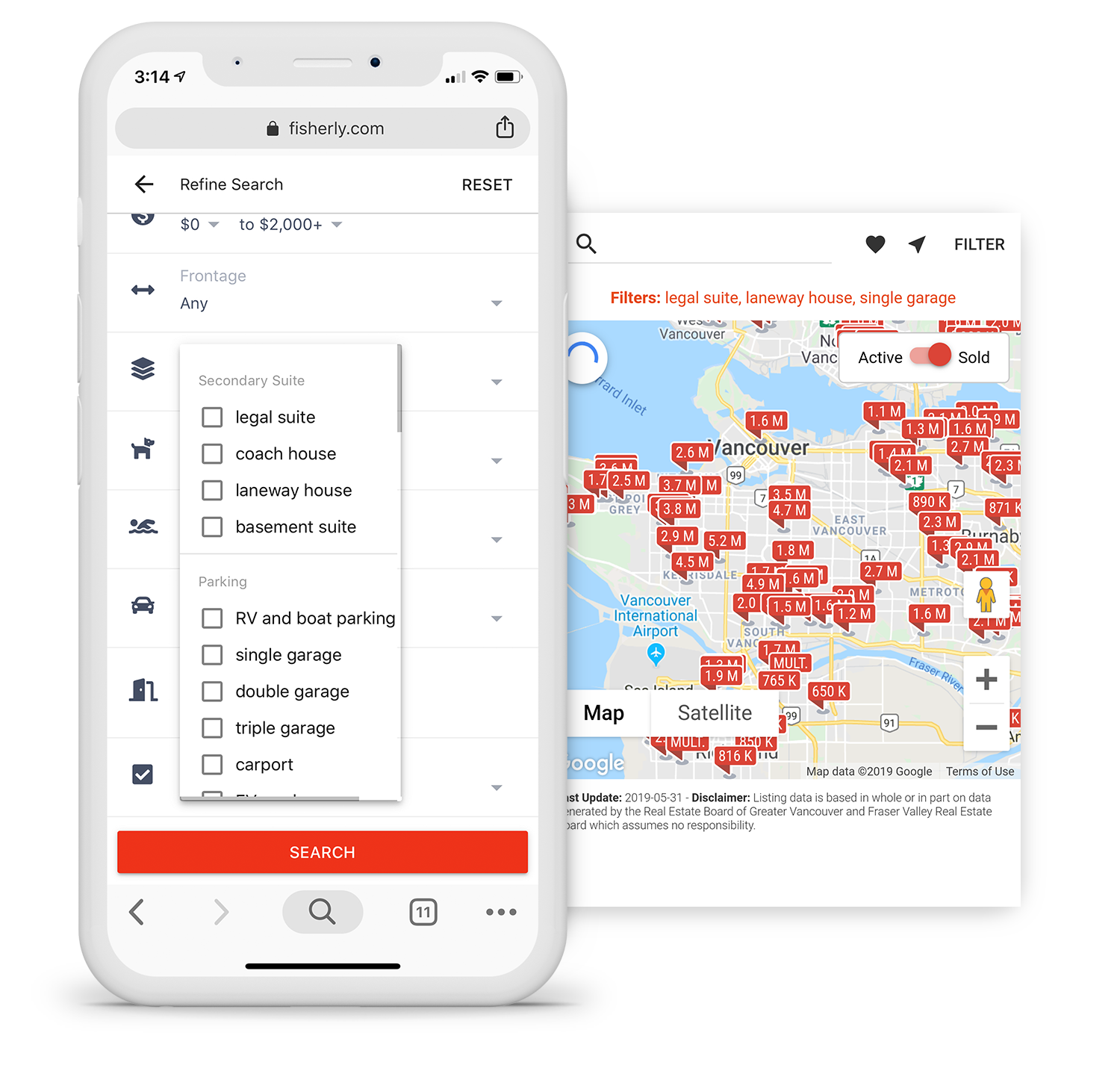The image depicts a smartphone application interface from Fisherly.com, designed to help users search for various types of residential properties with specific parking arrangements. The app allows searches for homes featuring a legal suite, coach house, laneway house, basement suite, and more. It includes a range of parking options such as boat parking, single garages, double garages, triple garages, and carports. On the right side of the image, there is a map showing locations in the Vancouver area that match the selected filters of a legal suite, laneway house, and single garage. Property prices in this listing vary widely, starting from around $650,000 and going up to $4.9 million, with an average property price of approximately $2 million. The interface is user-friendly and appears to cater to diverse housing needs and budget ranges.